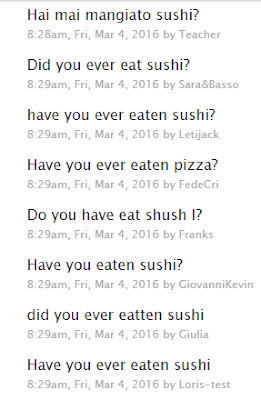The image features black text on a white background, containing a series of timestamped questions and statements about eating sushi. The text layout is as follows:

1. At the very top, the text reads: 
   "Hi My Mangiato Sushi"

2. Directly below this, another line reads:
   "8:28 AM Fri Mar 4, 2016 by Teacher"

3. The next entry reads:
   "Did You Ever Eat Sushi?"

4. Below, the timestamp is given as:
   "8:29 AM Fri Mar 4, 2016 by Sarah Ann Basso"

5. Another question follows:
   "Have You Ever Eaten Sushi"

6. The timestamp here is:
   "8:29 AM Fri Mar 4, 2016 by Letajack"

7. After that, it asks:
   "Have You Ever Eaten Pizza?"

8. The corresponding timestamp reads:
   "8:29 AM Fri Mar 4, 2016 by Fede Cry"

9. Next, another question appears:
   "Do You Have Eat Sushi?"

10. With the timestamp:
    "2:29 AM Fri Mar 4, 2016 by Franks"

11. Followed by another query:
    "Have You Eaten Sushi?"

12. The timestamp:
    "8:29 AM Fri Mar 4, 2016 by Giovanni Kevin"

13. Another question is included with a grammatical error:
    "Did You Ever Eaten Sushi" (with no question mark)

14. Followed by the timestamp:
    "8:29 AM Fri Mar 4, 2016 by Julia"

15. Reiterating a previous question without a question mark:
    "Have You Ever Eaten Sushi"

16. With the timestamp:
    "8:29 AM Fri Mar 4, 2016 by Loris Dash Test"

The background is white, with the text primarily in black. However, the timestamps and author names are in a darker gray color, creating a subtle contrast.